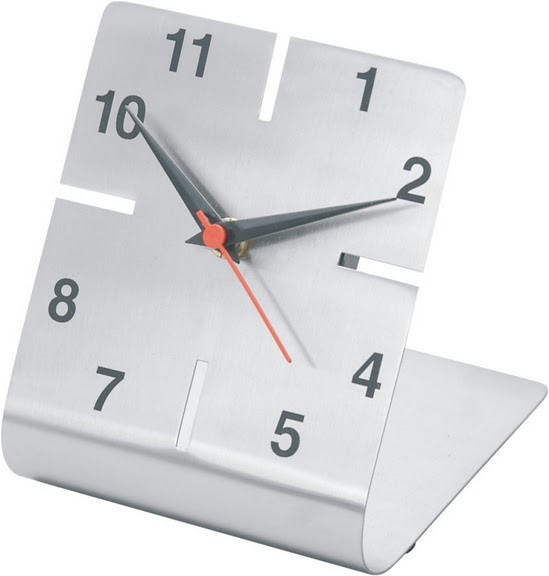The image features a uniquely designed clock set against a stark white background. The clock’s structure resembles a bent rectangle, laying flat at the bottom and curving upwards towards the front. Its face is minimalist, adorned with a smattering of numbers: 1, 2, missing 3, 4, 5, missing 6, 7, 8, missing 9, 10, 11, and missing 12. These missing numbers are marked by indentations or empty rectangular spaces, creating a striking visual pattern. The hour and minute hands are black, while the second hand stands out in red. The time displayed is 10:10.